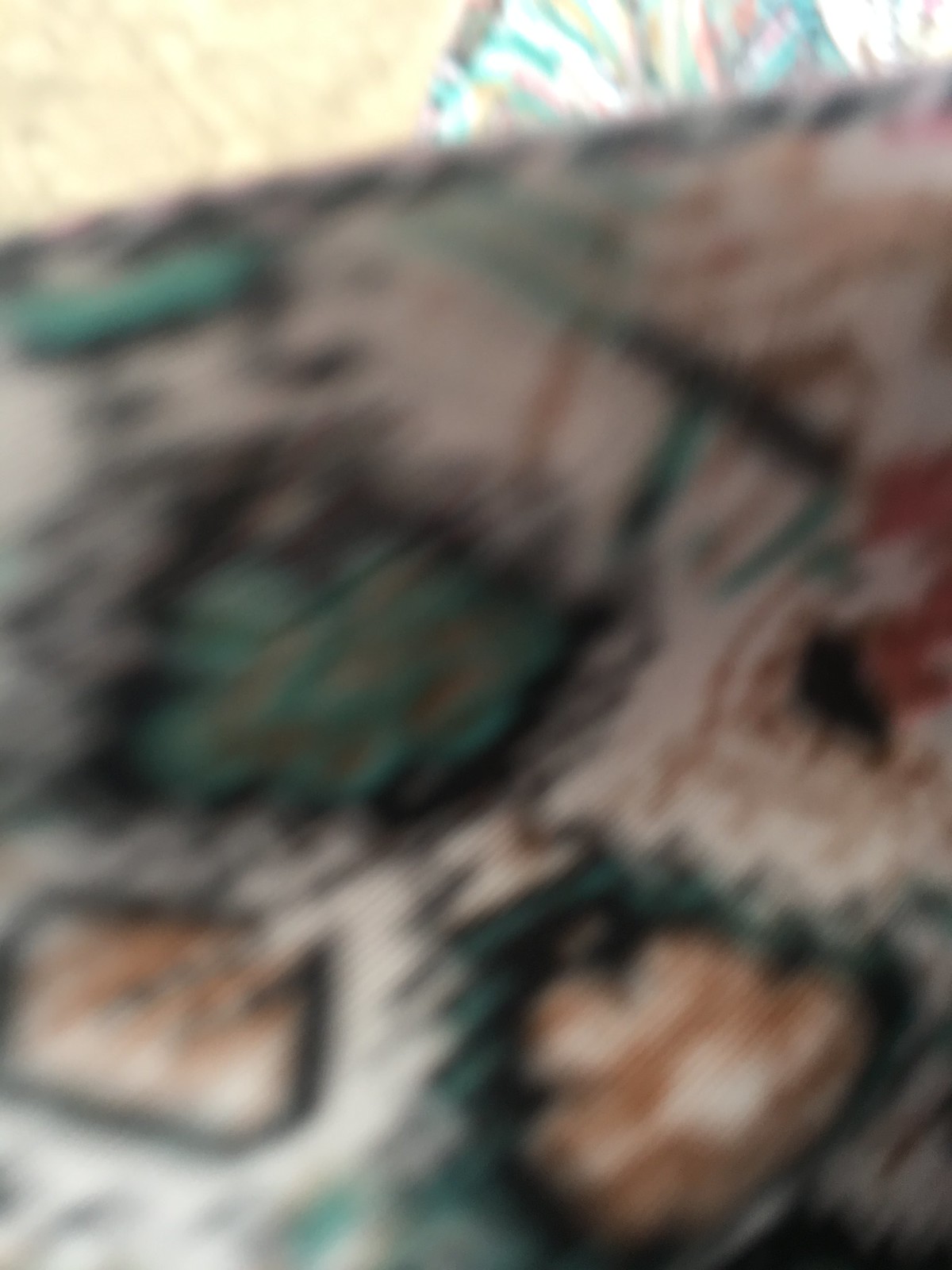This image depicts an out-of-focus wall adorned with various forms of graffiti or artwork. The wall predominantly features a white background. Towards the lower right corner, there are intricate images rendered in tan or light brown with white accents, all encased in a dark outline and complemented by a shade of green.

On the lower left portion of the image, there is a stylized capital letter "G" in black, filled with brown details on the inside. Near the center left, a shape resembling a Christmas tree, painted in green and outlined in black, stands out prominently.

Additional brown shapes and lines are scattered on the upper right-hand section of the image. The top portion of the wall appears to be delineated by a black outline, with hints of green on the lower left side of this top margin. The background at the top left exhibits a tan color, while the top right side showcases a blue and white object, adding to the eclectic nature of the mural.